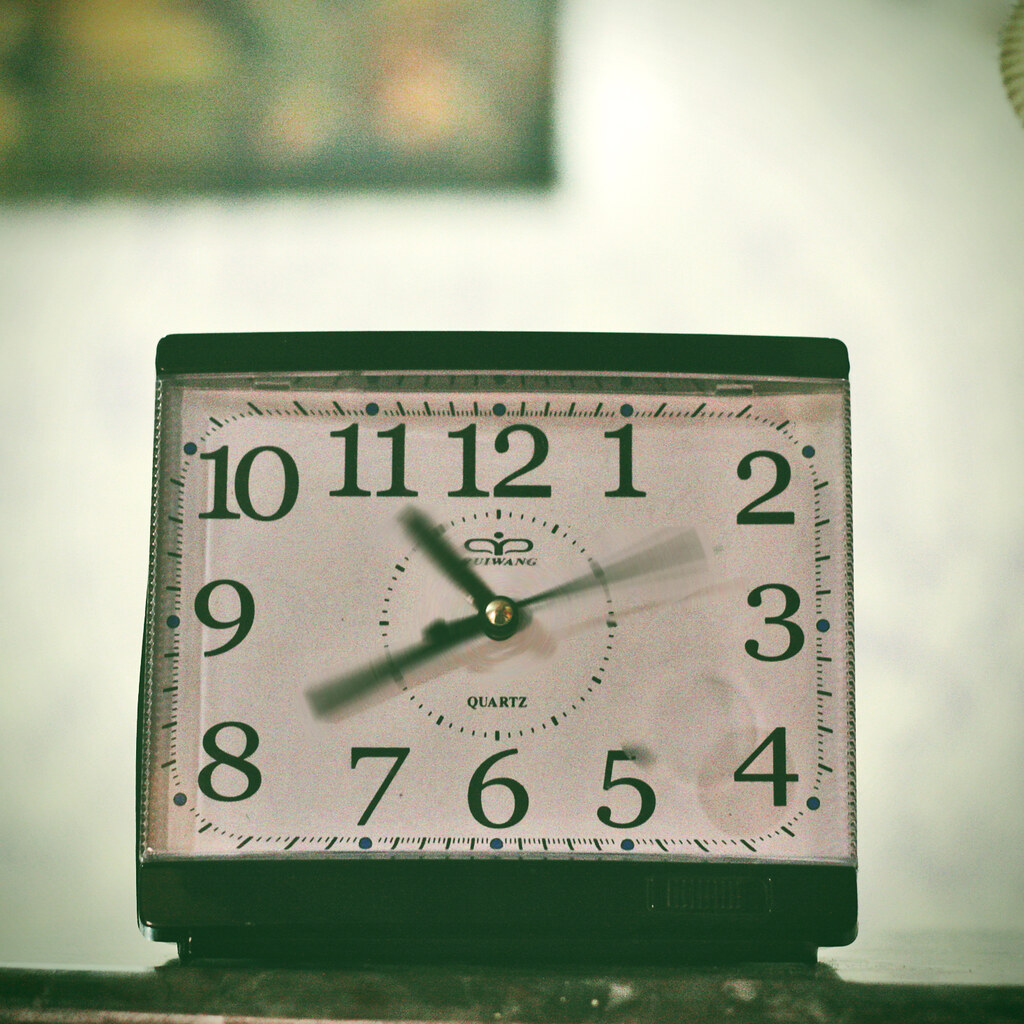The photograph showcases a vintage-style, rectangular clock centrally placed against an off-white wall. The clock, roughly 8 by 8 inches, is characterized by its rectangular face with an unconventional arrangement of numbers. The numbers 11, 12, and 1 are aligned in a row at the top, while the numbers 2, 3, 4 on one side and 8, 9, 10 on the other create vertical lines, and the numbers 5, 6, 7 are straight at the bottom. The clock, positioned on a black surface, features a minute hand pointing at 11, an hour hand at 8, and a second hand at 2. All three hands are captured in motion, appearing blurry, which contrasts with the otherwise sharp image of the clock itself, suggesting a long exposure. The clock face has a grainy, whitish-pink tint, and a brand name with a logo that includes the word "Quartz." The image has a bluish-yellow tint, adding to its artistic vintage aesthetic. A blurred painting or illustration is faintly discernible in the upper left corner of the background, adding a subtle depth to the scene.